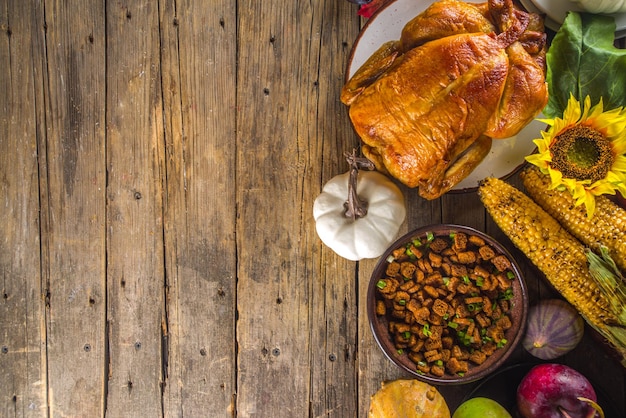In this vibrant photographic image capturing a quintessential Thanksgiving meal, the left-hand side of the wooden table remains empty, showcasing rich, brown wood grains, while the right-hand side brims with a feast of autumnal delights. From a bird’s eye perspective, we see a cooked golden turkey on a white plate at the top right. Surrounding the turkey, a colorful array of gourds in hues of green, purple, white, yellow, and orange populate the scene, including a small white gourd at the turkey's lower left. A cheerful, sunny yellow sunflower with green leaves is positioned to the right of the turkey, adding a touch of brightness. Below the sunflower, two ears of roasted corn angle out of the frame, nestled beside a red onion at the bottom right. A bowl filled with what appears to be stuffing, resembling tiny brown bits, sits close to the onion. Completing the festive spread, a yellow squash lies below the bowl. The harmonious autumn-themed color palette and meticulous arrangement of elements invite viewers to celebrate the warmth and abundance of Thanksgiving.